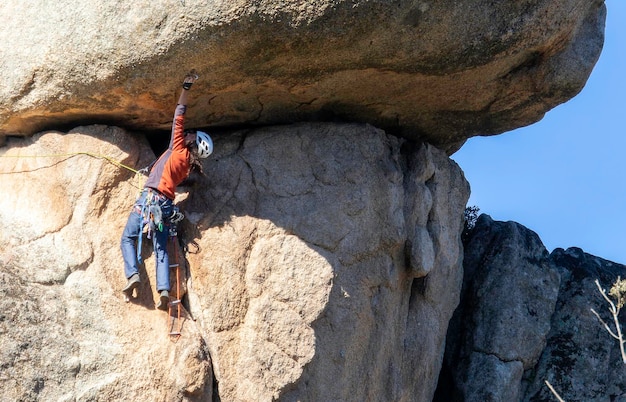The image depicts a rock climber scaling a steep rock face beneath a prominent overhanging outcrop. The climber, dressed in blue jeans and an orange and purple long-sleeved shirt, is outfitted with a white helmet and gray shoes. He is secured with a yellow-green belay rope that extends to the left side of the frame. His left hand is reaching up to hook into the rock wall, while various climbing gear, including an orange ladder-like piece, dangles from his waist. The scene is set against a backdrop of clear blue sky and a scraggly tree visible on the right side of the picture, lending additional context to the rugged environment.